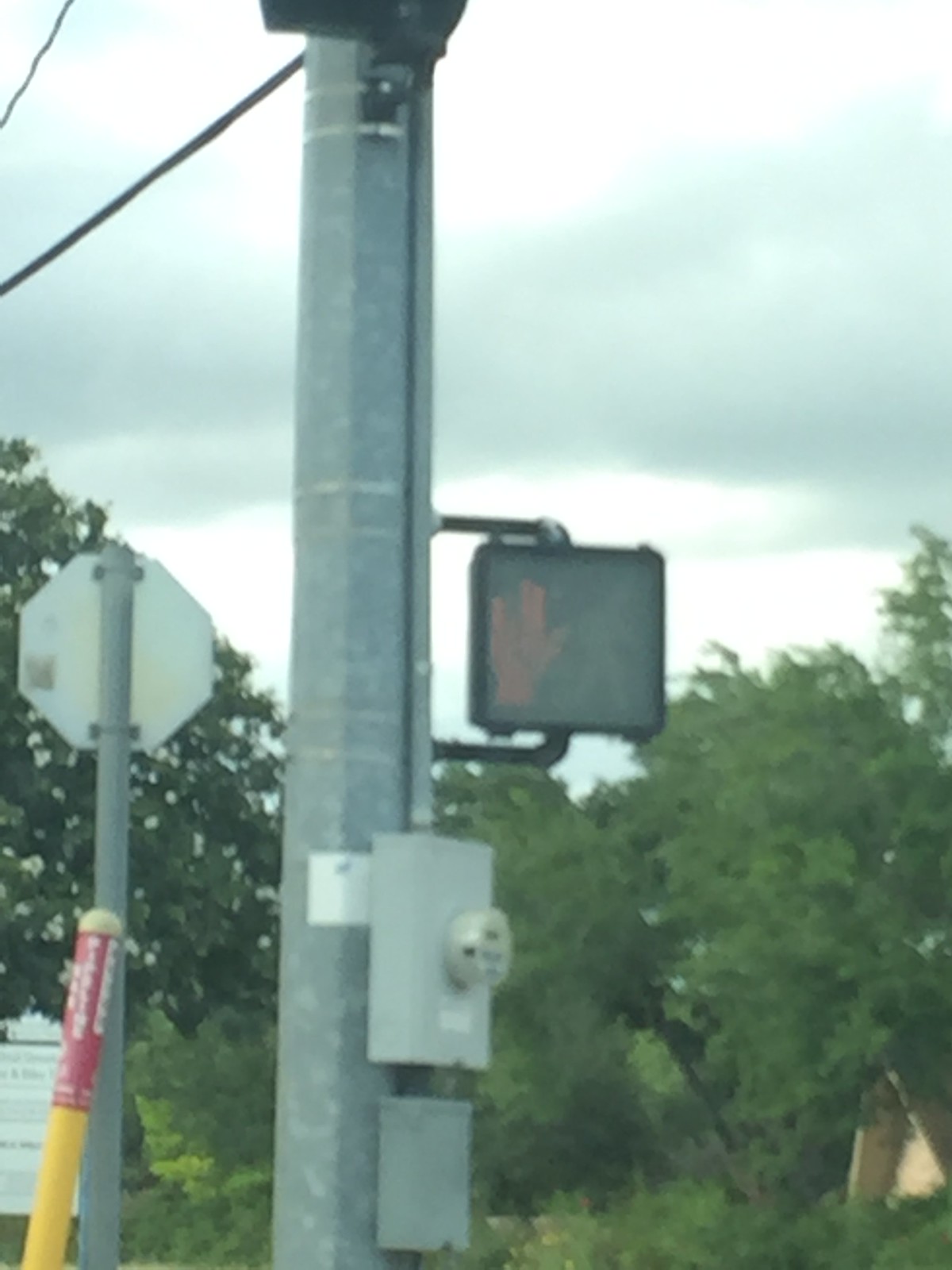The image portrays a bustling urban intersection dominated by a pedestrian traffic light mounted on a thick metal pole. The pedestrian signal features a lit red hand, signaling pedestrians to stop, and is flanked by utility boxes—one with a visible meter—attached to the same pole. To the left of this setup, the gray backside of an octagonal stop sign on its own metal pole is seen. In the foreground, a short yellow pole wrapped with red paper and thick white lettering stands out, next to a small white sign with black writing that's too distant to read. The scene is framed by a backdrop of tall trees and a yellow house partially obscured by the foliage. The sky is overcast, laden with thick clouds, hinting at impending rain.